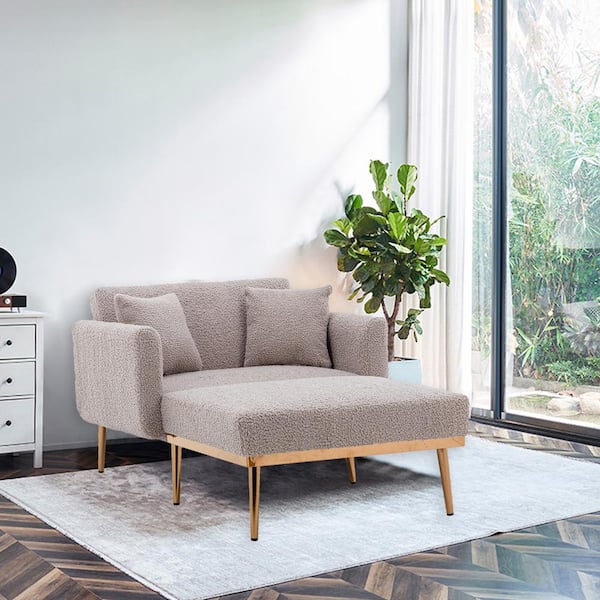This image depicts a detailed 3D color-rendered living room scene with a square format, likely created using an app like SketchUp. The room has light white walls with a possible tint of blue or green. Prominently featured is a plush, gray two-seat love seat with matching fabric, complete with two stuffed pillows. The love seat has an integrated ottoman extension, producing a chaise lounge effect with four brass legs. The furniture arrangement sits on a gray rug, which lies atop a dark to medium brown herringbone wood floor.

To the right of the love seat, there is a tall green plant, likely a four-foot-tall palm-leaf variety in a white container. Adjacent to the plant are floor-to-ceiling sliding glass doors that allow ample sunlight to flood the room, casting light on the plant and revealing an outside garden area. A sheer white curtain hangs on the left side of the doors.

To the left of the love seat is a small, white three-drawer chest of drawers with a decorative knickknack placed on top. The entire composition of the room, including the parquet flooring, the chic modern furniture, and the serene view outside, suggests a cozy yet stylish living space.